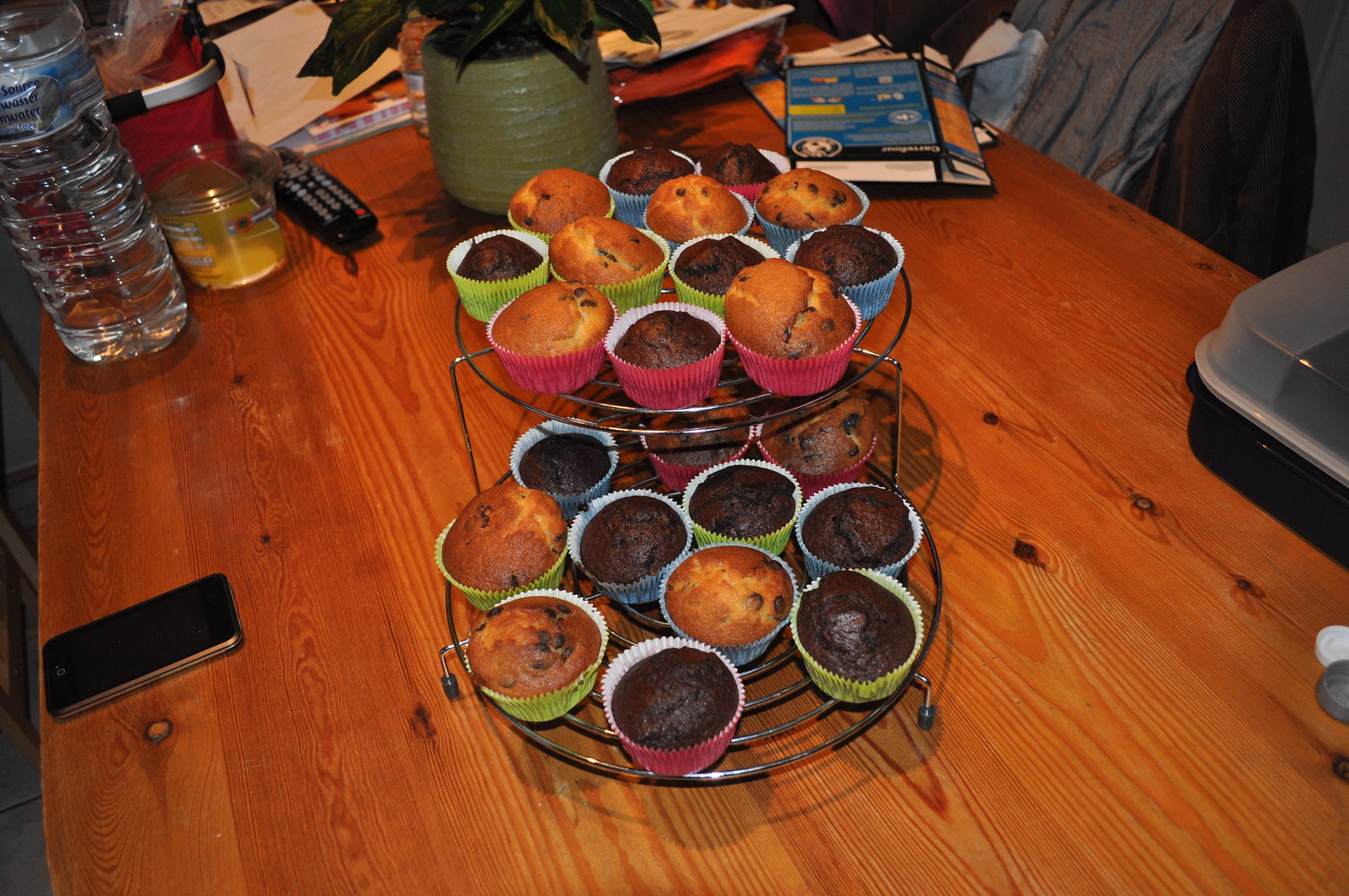The image shows a two-tiered dark metal wire rack filled with a variety of muffins and cupcakes, displayed prominently in the center of a rustic, reddish wooden table with visible knots, reminiscent of a picnic-style bench. The baked goods are in colorful paper cups—green, pink, and blue—and include both dark brown chocolate and lighter chocolate chip muffins. Surrounding the rack, various items clutter the table, including a cell phone to the left, a water bottle, a green ceramic pot with a succulent plant, a candle, multiple boxes and containers, a remote, and a black Tupperware container with a clear top on the right. The scene appears to be set in a kitchen, giving a cozy, homemade feel to the setting.